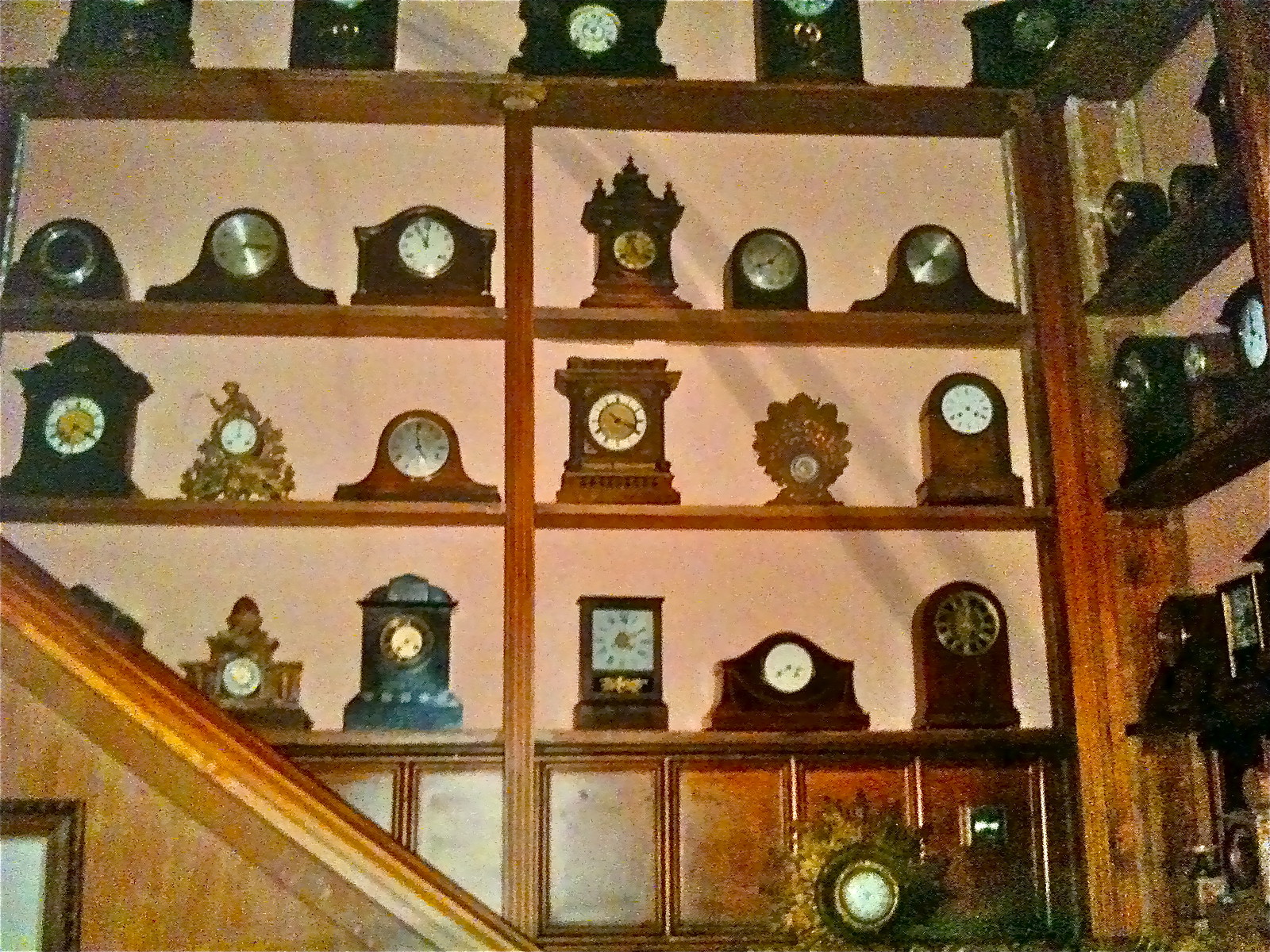The image appears to be a slightly grainy, vintage photograph of a stairway corner in someone's home or a clock collector's space, featuring an extensive collection of old-fashioned mantel clocks. The scene includes a staircase with a wooden handrail visible in the bottom left corner, ascending from the bottom center to the middle left of the image. Surrounding the stairs, a series of wooden shelves form an L-shape, lined with an array of over 30 different tabletop and mantel clocks of various shapes, sizes, and designs. The shelves, reminiscent of bookcases, hold clocks that range from round and square to arched and pointed, resembling castle fronts. The clocks predominantly have wooden frames, with some featuring brass and gold accents. The clock faces vary in color and design, including white, metal, and gold. The shelves themselves are worn, contributing to the vintage feel of the space, which includes a backdrop of light pink or beige walls. None of the clocks show the same time, suggesting they might be non-functional or simply not synchronized. Overall, the image captures the essence of a dedicated clock collector's display, rich with historical and aesthetic charm.